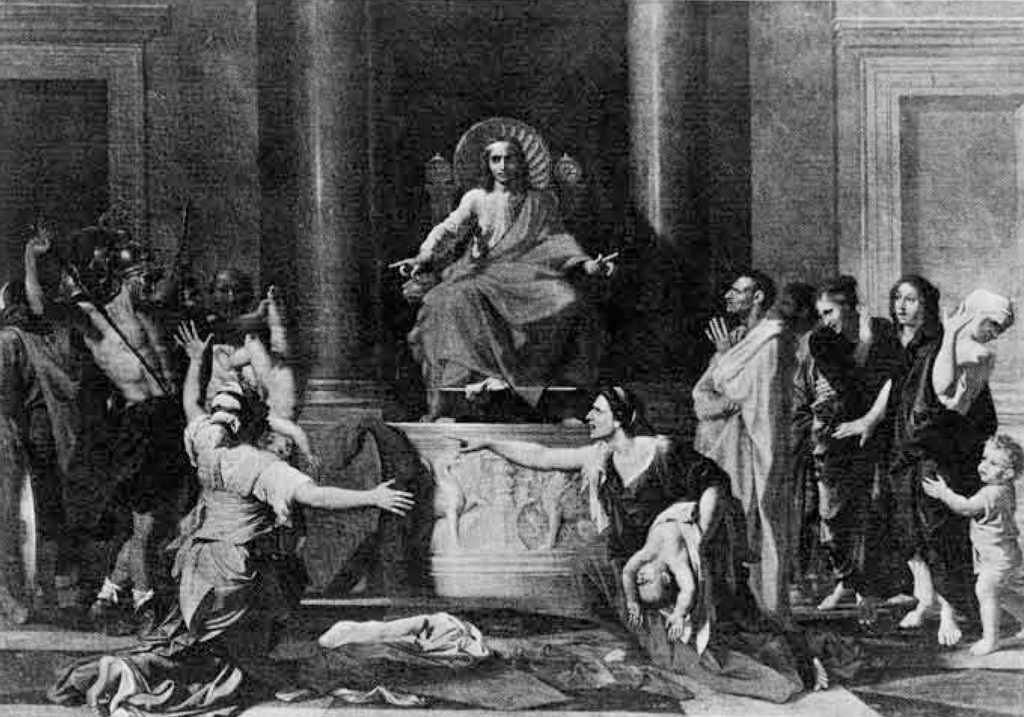In this renowned black and white depiction of the Judgment of Solomon, a pivotal moment from biblical lore is brought to life with striking emotional intensity. At the center of the image is King Solomon, seated on his throne, exuding authority and wisdom. Draped in a majestic robe that covers one shoulder, Solomon points towards both sides, commanding the scene.

In the foreground, the dramatic tension is palpable. Two women kneel—one cradles a draped child, who appears to be either asleep or unconscious. Her expression is resolute, contrasting sharply with the other woman, whose arms are outstretched in a gesture of profound grief and desperation, her face contorted with anxiety or surprise. This stark juxtaposition captures the essence of their heart-wrenching dispute.

Flanking the women, onlookers stand with hands raised, turning away as if overwhelmed by the intensity of the situation. The textured garments and drapery spread across the floor add layers of realism and depth to the scene. Solomon’s judgment is set against a backdrop of imposing pillars, enhancing the gravity and solemnity of the moment.

This emblematic image, often referred to as “Solomon’s Ordeal,” masterfully conveys the raw emotion and moral gravitas of the legendary tale, making it an enduring symbol of wisdom and justice.